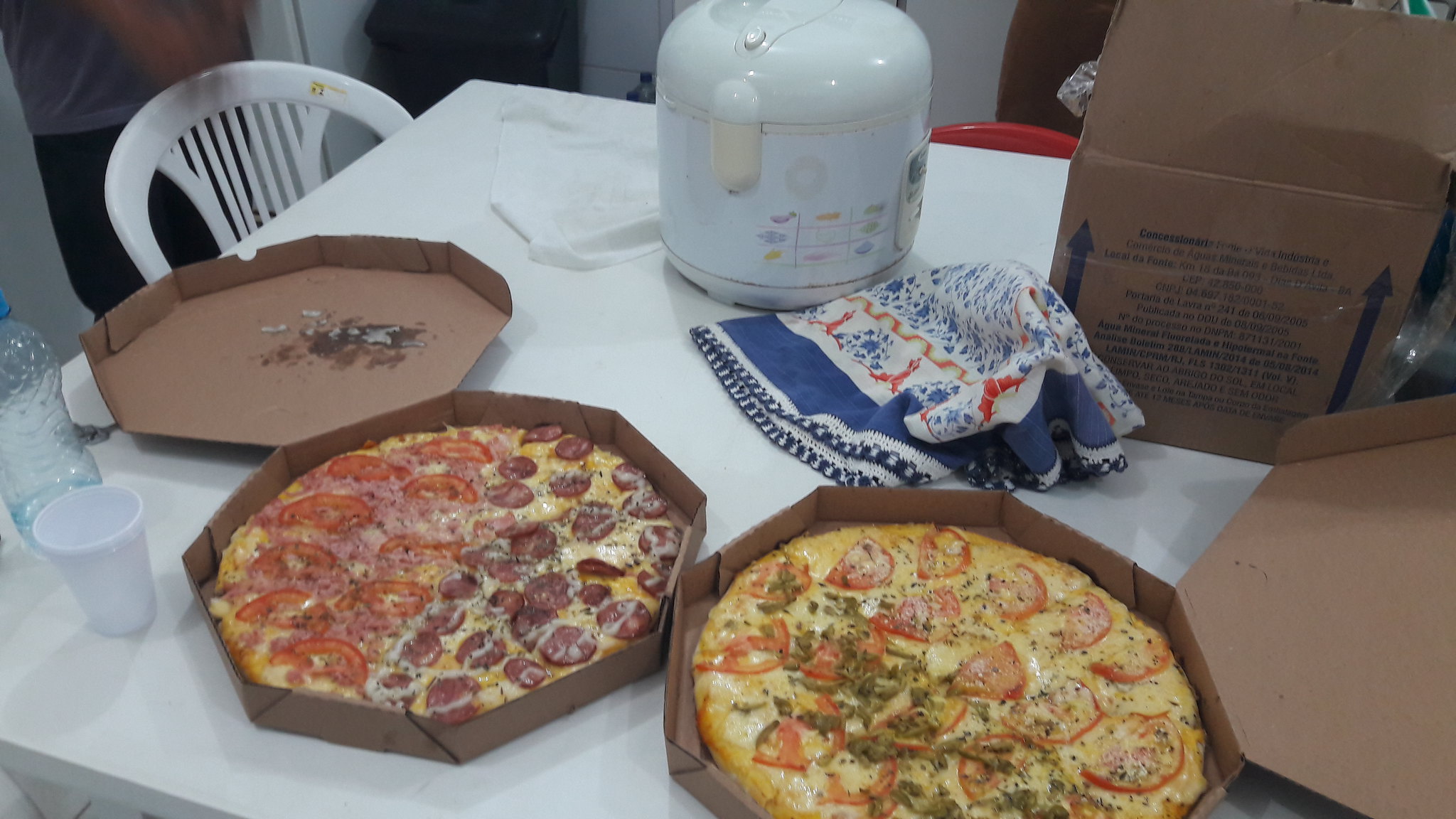This photograph showcases a white plastic table, typically used outdoors but placed inside a house, distinguished by glimpses of walls and doors in the background. Prominently displayed on the table are two open, hexagonal pizza boxes. The pizza on the left features a variety split between halves: one side topped with cheese and tomatoes, garnished with greens, and the other adorned with circular slices of either pepperoni or salami. The right pizza also presents a mix: one half is primarily cheese and tomato, with possible jalapeño pieces, while the other side suggests a similar mix of toppings. Additional items on the table include a blue and red kitchen towel, a white cup, an empty water bottle, and a large white container, possibly a pressure cooker or small propane tank, housed in a cardboard box. At the back of the table, a white plastic chair, typically used for outdoor seating, completes the scene.